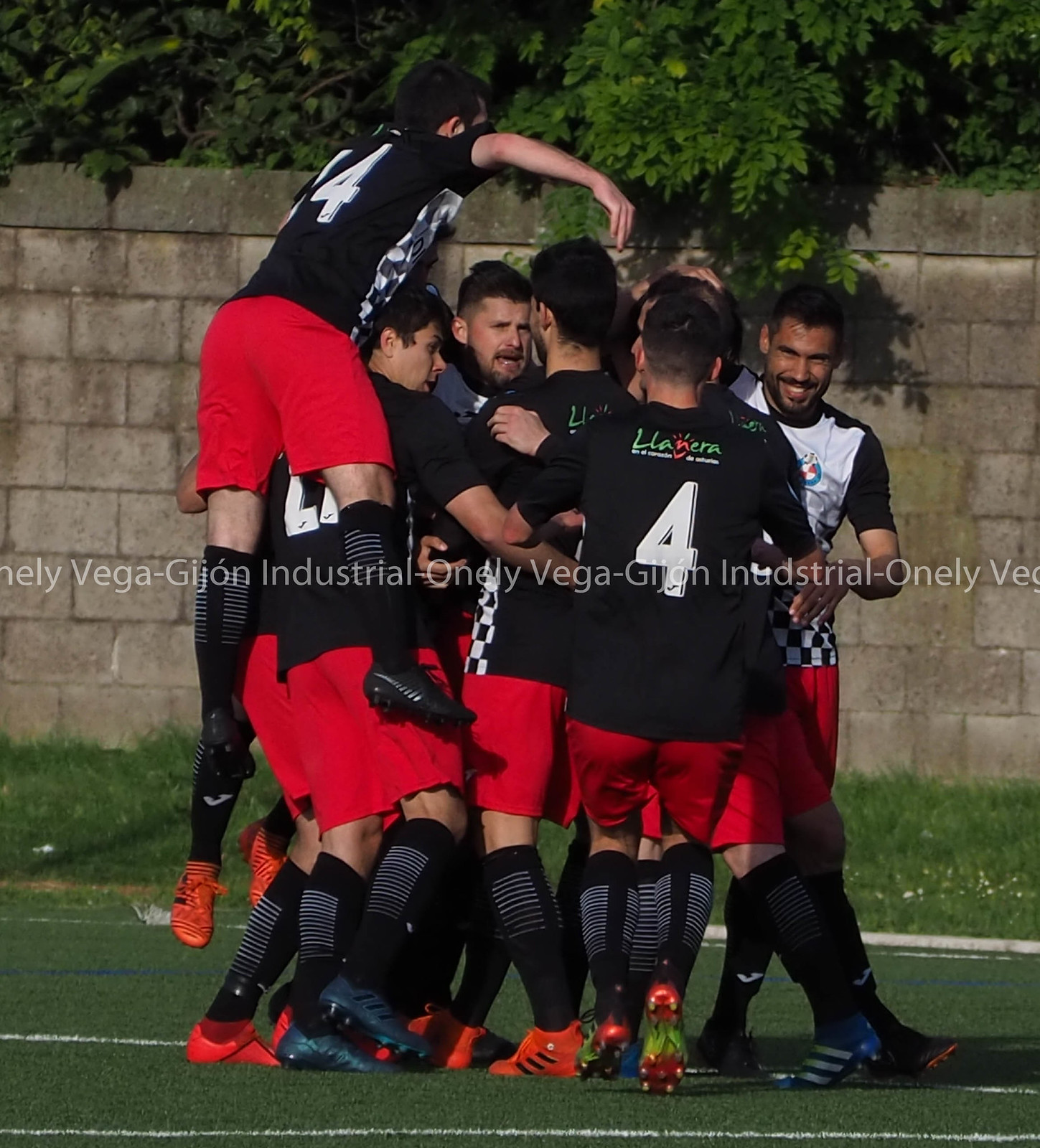The image depicts a celebratory scene on a soccer field, with green grass and white lines indicating the pitch. In the center, a group of men are tightly huddled together, seemingly in exuberance, likely after scoring a goal. Emphasizing the moment, a man on the left is captured mid-air with arms outstretched above the group. The players are donning black jerseys with white numbers, specifically with the numbers 4 and 14 visible. Additionally, their attire includes red shorts and knee-high black socks with white stripes. Footwear varies, with most players in black cleats, though some are wearing red, blue with white stripes, and grayish black Adidas cleats. A repeating watermark, "Only Vega Gijon Industrial," is superimposed across the image. The background features a gray cinder block wall, hovering greenery, and shrubbery above the wall.